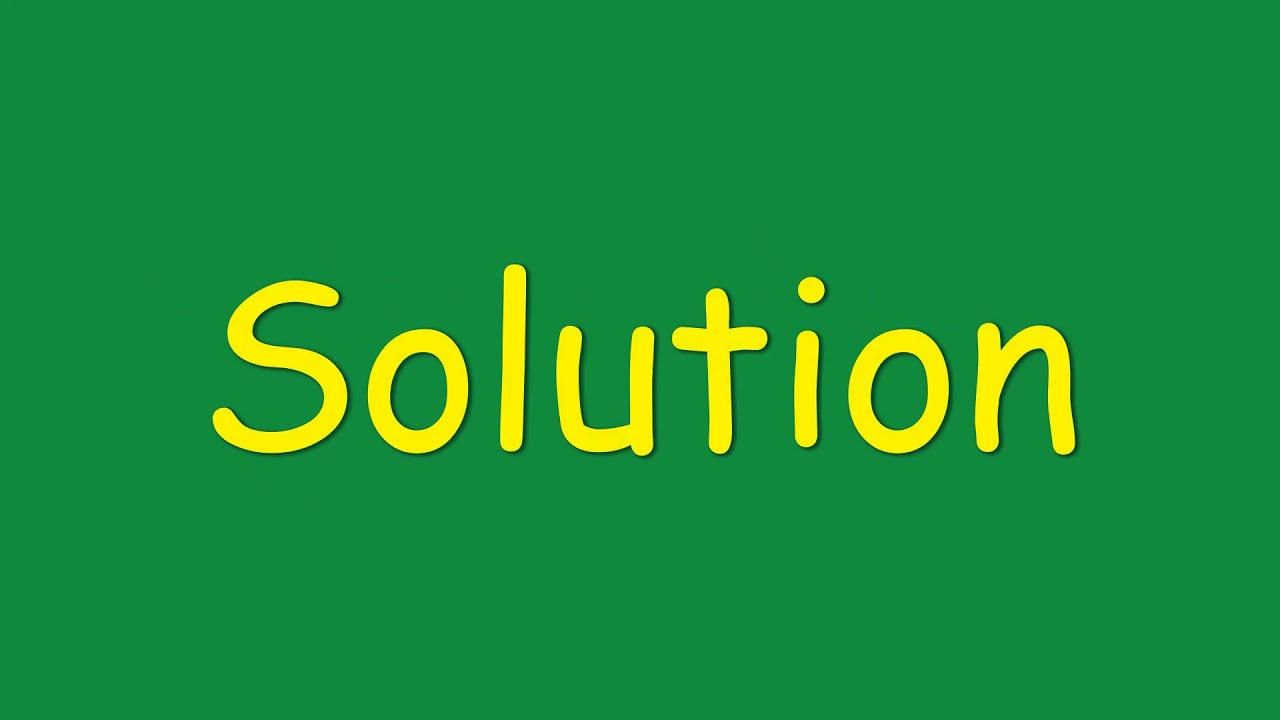The image features a landscape-oriented rectangle with a green background and the word "Solution" prominently displayed in the center. The text, written in a playful handwritten font, begins with a capital 'S' followed by lowercase letters. The word is filled with a vibrant yellow color and slightly spaced out, giving it a non-serious appearance. The letters cast subtle shadows on the green background, creating a faint shadow effect. The width of the image is approximately 1.5 times its height. There is a barely noticeable green outline around the yellow lettering, enhancing its visibility against the green backdrop.